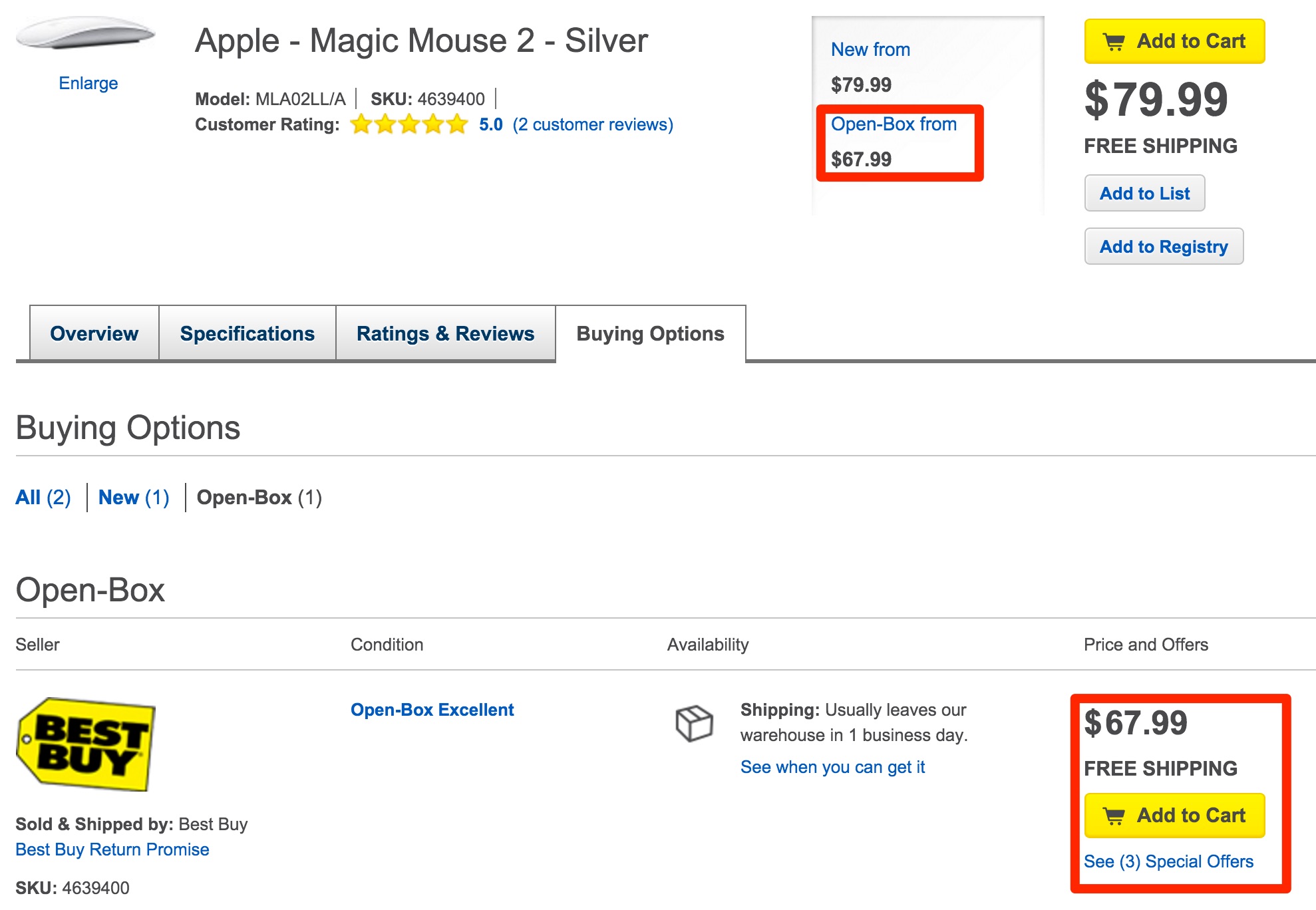A screenshot of a Best Buy webpage depicts a search for mice, specifically highlighting the Apple Magic Mouse 2 in Silver. The product is prominently displayed with prices listed: new for $79.99 and open box for $67.99. The open box price is emphasized with an outline around it, appearing both near the product image and in a lower section where the buyer can choose between new and open box options. Additional navigation tabs—'Buying Options', 'Ratings and Reviews', 'Specifications', and 'Overview'—are visible, showcasing a detailed layout for potential buyers. The background is primarily white with occasional yellow accents and the recognizable Best Buy logo. The product has a five-star rating based on two reviews.